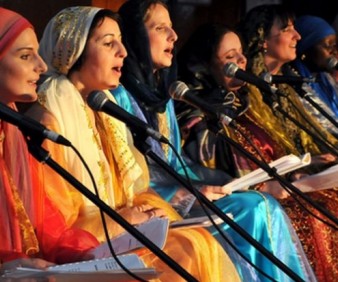This painting depicts a close-up scene of six women seated in a row, all facing towards the right. Each woman is adorned in long, brightly colored pastel dresses and head coverings that match their outfits, signifying a potential cultural or religious context. The colors of their attire range from red and yellow to teal, orange-yellow, darker red, darker yellow, and blue as they recede into the background. Positioned in front of each woman is a microphone on a stand, angled in from the bottom right of the image. Musically themed, each woman holds sheet music on her lap, suggesting they might be singing, as indicated by their lip movements. Most of the women appear to be vocalizing, while others are simply smiling, adding to the harmonious ambiance of the scene.